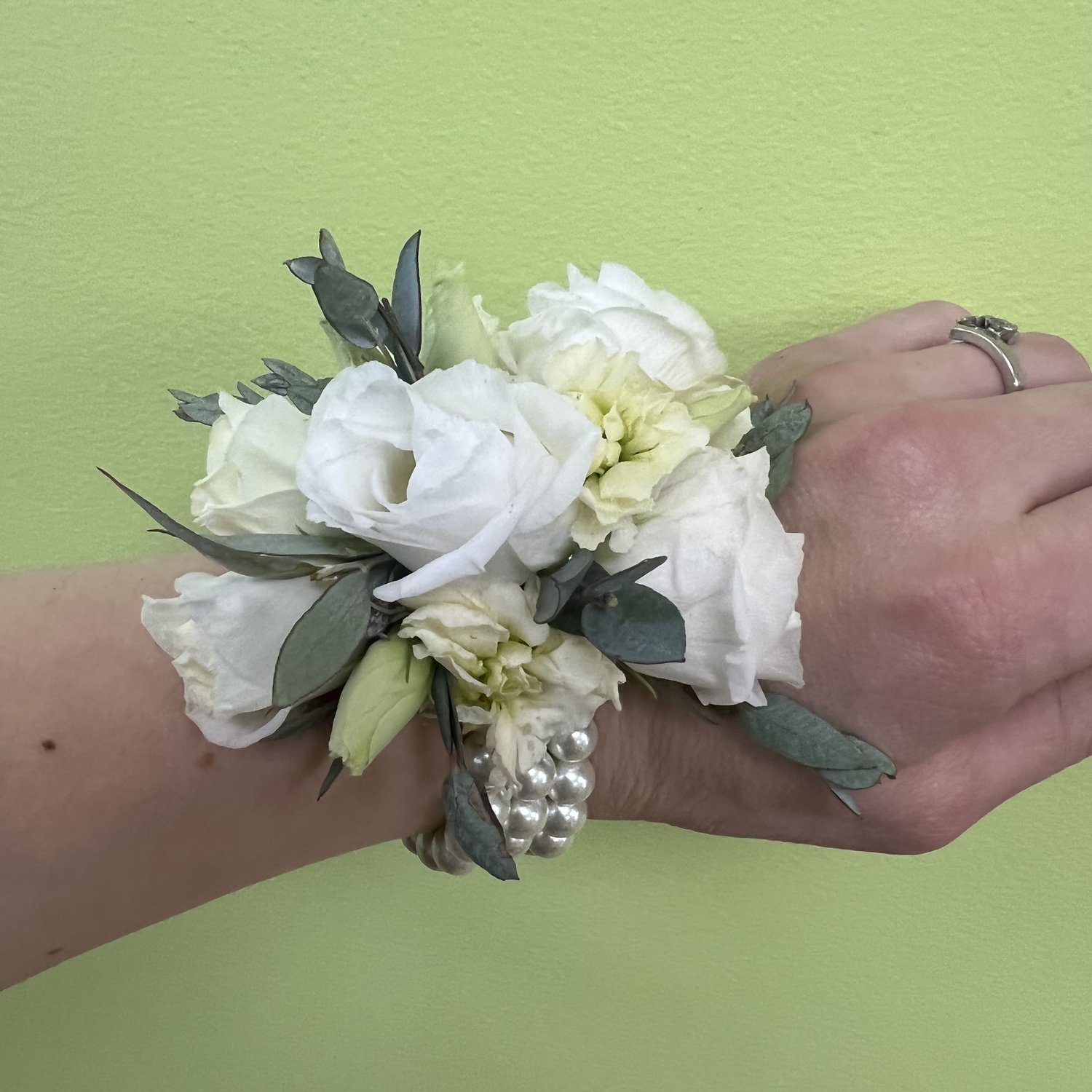This close-up photograph features a woman’s left hand adorned with intricate details. Her hand, resting against a bright lime green background, showcases a silver ring with a designed precious stone on her ring finger. The wrist is elegantly decorated with a corsage composed of both closed and open white roses, accompanied by two other small white flowers and green foliage peeking through. The corsage is festooned onto a triple-stacked pearl bracelet, adding to the sophisticated charm. Additionally, there are green branch stems that enhance the floral arrangement, making it a probable accessory for a special occasion like a dance or a prom.